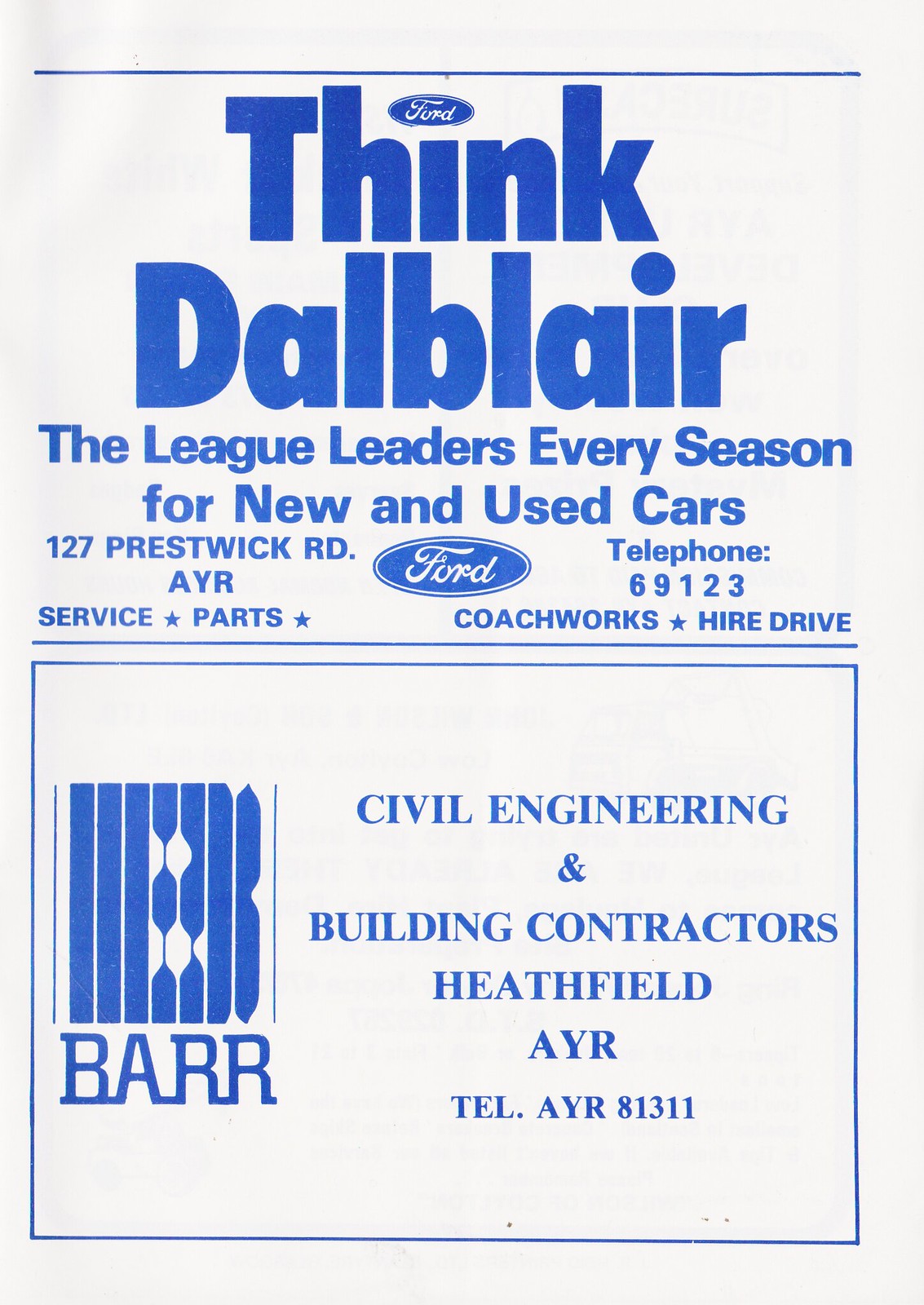This image is a scan from a magazine, specifically the right side of a folded page, suggested by visible creases in the upper left corner and the faint bleed-through of an image from the opposite side. The page features a white background with blue printing, illustrating two advertisements. 

In the upper half, there’s a prominent advertisement for Dalblair, highlighted by the large, bold headline "Think Dalblair." The ad markets the business as "the league leaders every season for new and used cars" and provides their address, "127 Prestwick Road, Ayr." There is a Ford logo included, and beside it, the text "Telephone 69123." At the bottom of this ad, services such as "Service Star Parts Star" are delineated on the left and "Coach Works Star Hire Drive" on the right.

Below this, there is another ad encased in a thin blue-lined box. This is for a company labeled "Bar" with a unique logo composed of vertical slats forming the letter 'B'. Adjacent to this, the ad identifies the business as "Civil Engineering and Building Contractors." Further information includes their location at "Heathfield, Ayr" and the telephone number "Ayr 81311."

This scan likely originates from a football match program (soccer, in the US context), given the dual advertisements and simple, monochromatic blue on white layout.